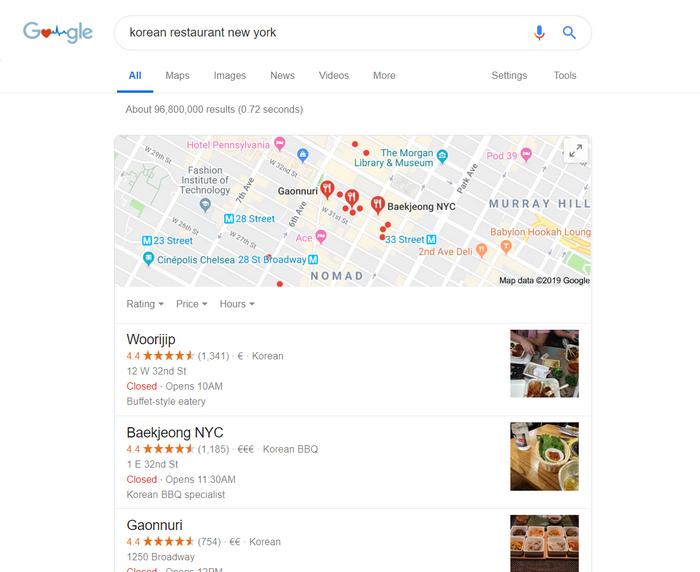This image depicts a Google search results page, prominently featuring the Google logo in the top left corner. The page is themed in celebration of heart health awareness, evidenced by a heart icon accompanied by an animated heartbeat line.

The search query entered in the bar is "Korean restaurants New York," with a microphone icon available for voice search. The results indicate approximately 96,800,000 entries found in 0.72 seconds. Below the search bar, standard Google navigation options such as All, Maps, Images, News, Videos, More, Settings, and Tools are visible.

A map highlights several local landmarks and selected Korean restaurants in New York City. Details of three restaurants are provided:

1. **Woorijip** - Located at 12 West 32nd Street, this restaurant is known for its affordability and has a rating of 4.4 stars based on 1,341 reviews. It is currently closed and will reopen at 10 a.m.

2. **Baekjeong NYC** - Situated at 1 East 32nd Street, Baekjeong NYC is a pricier option with a specialty in Korean barbecue. It holds a 4.4-star rating from 1,185 reviews. The restaurant is closed and scheduled to reopen at 11:30 a.m.

3. **Gaonnuri** - This mid-priced Korean restaurant can be found at 1250 Broadway. It has a 4.4-star rating with 754 reviews. Gaonnuri is currently closed and will reopen at 12 p.m.

The screenshot is sufficiently large, suggesting it may have been taken from a tablet or small laptop rather than a mobile device. This detailed display of Google search results illustrates a user's quest to find a Korean restaurant in New York City.